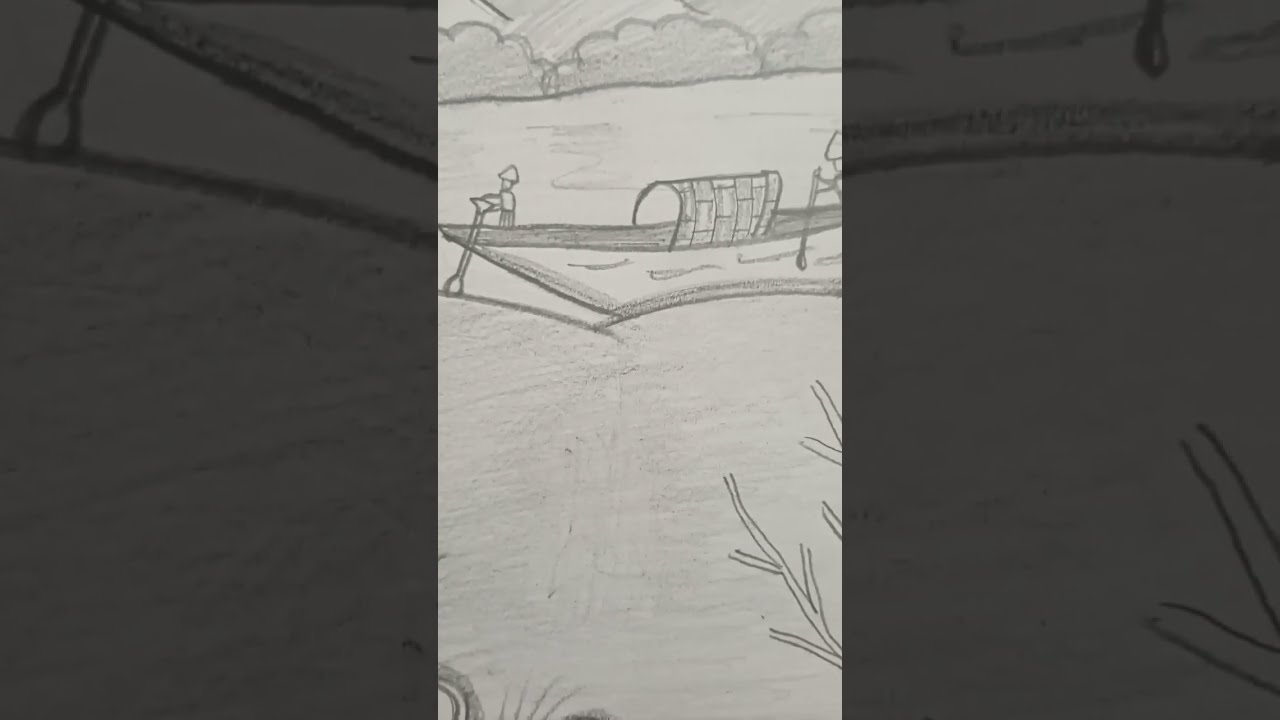This image features a detailed pencil drawing presented in a triptych format, with the left and right panels slightly darkened to highlight the central panel. The central focus is a brightly lit, zoomed-in section of the artwork. The drawing portrays a long boat on a body of water, flanked by two individuals wearing hats standing at the boat's bow and stern, each rowing with long oars from the same side, giving the impression they might be moving in circles. The boat includes a covered structure in the middle, resembling a tunnel or shaded area. The background showcases a simple, child-like depiction of foliage and trees, with a hint of a distant shoreline, while the foreground features scribbled land with branches, plants, and possibly flowers extending from the right and left corners, adding depth and texture to the scene.